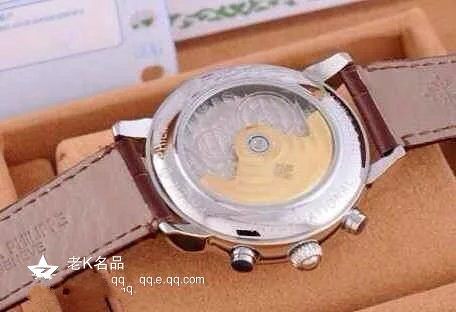The photograph prominently features a silver wristwatch with brown leather straps, encased in an ornamental, rusty orange-brown display box, positioned centrally. The watch face exhibits distinctive color variations, including an eye-catching beige light brown area in an unconventional shape. In the background, there is a soft blur of gray and white documents, one of which has a green border. Subtle yet visible lettering and a non-English website are present in the lower right-hand corner of the image, adding an additional layer of complexity to the scene.